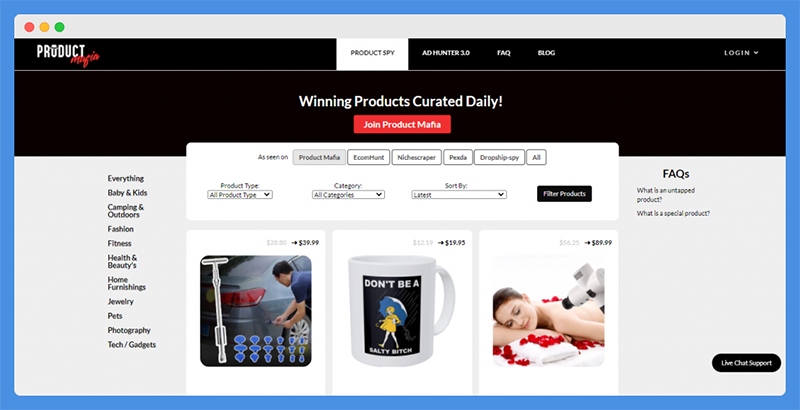This image, taken from a website, features a bordered layout with a light blue border of about a quarter-inch width surrounding the entire photo. At the top, a light gray strip also measures around a quarter-inch in height. Positioned in the top-left corner are three circles: red, yellow, and green, reminiscent of traffic lights. Below this top section is a black border approximately half an inch thick, followed by a thin white line, and then another segment of about two inches of black border.

In the upper portion of the black border, bold white text spells "PRODUCT," and directly below that, the word "Imagine" appears in red. Centrally located within this black border is a white tab labeled "PRODUCT SPY" in black text. Adjacent to it are several navigation options in red text: "WHAT," "FAQ," "BLOG," and on the far right, a "LOGIN" option with a drop-down tab.

Beneath the "PRODUCT SPY" label, bold white text announces "WINNING PRODUCTS CREATED DAILY." Below this proclamation, a red tab houses white text that reads "JOIN PRODUCT MAFIA."

On the left side of the page, beneath these elements, the background is a light gray featuring a list of clickable categories, including "Baby Gifts," "Camping Outdoors," "Fashion," and several others. On the right side, there is another section labeled "FAQs" with two clickable questions underneath.

Centrally located, between the left and right sections, is a large white square. At the top of this square, the text "AS SEEN ON" is displayed, accompanied by six tabs; one is gray while the others are white with black lettering. Below this area, there are three drop-down tabs: "Product Type," "Category," and "Sort By." To the right of these tabs is a black rectangle featuring "Filter Products" in white text.

Finally, below this entire arrangement, the product display area showcases three purchasable items. The top right corner of each item’s picture displays its price. The first product on display appears to be a tire jack for a car, showing the rear end of a car next to a man. The second product is a mug adorned with the Morton Salt Shaker person, and the third product illustrates a woman receiving a massage.